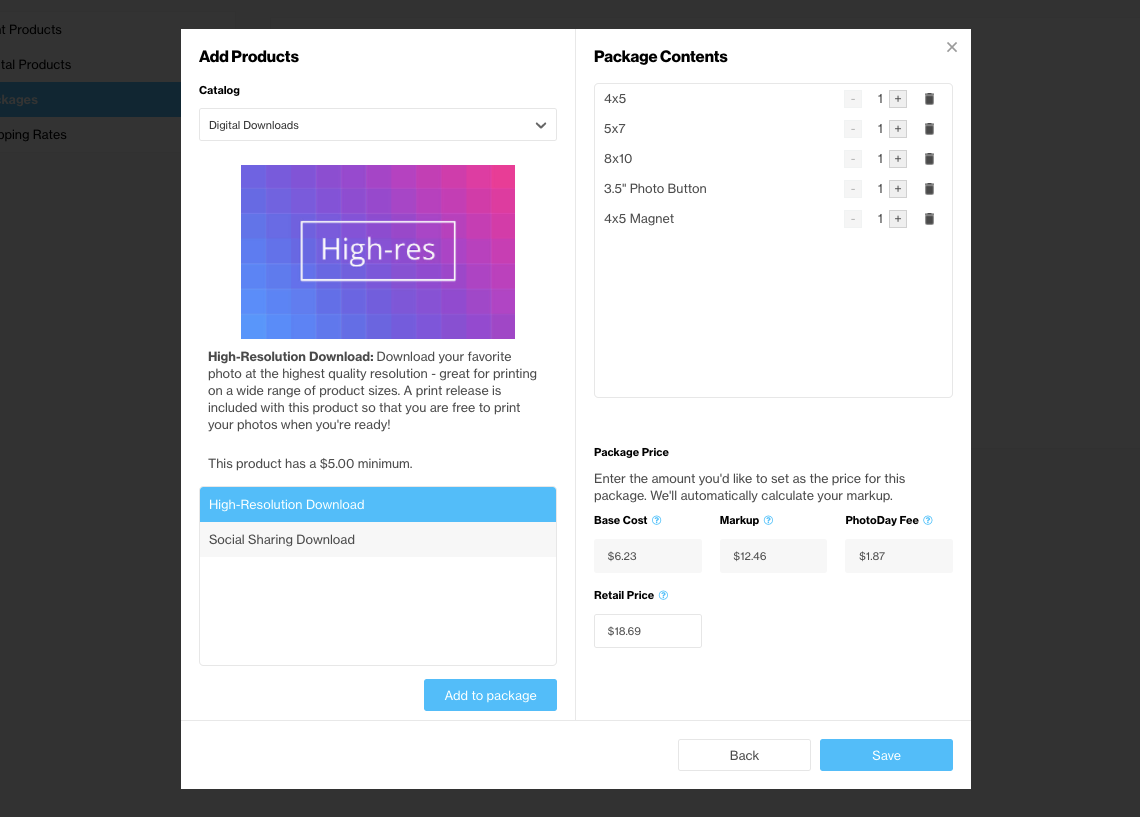The image depicts a detailed view of a shopper's digital cart on an e-commerce platform, specifically at the checkout stage for purchasing digital media and print products. The screen is divided into two sections:

On the left side:
- At the top-left corner, there's an "Add Products" heading, under which "Catalog" is listed.
- The user has selected the "Digital Downloads" category.
- The primary option displayed is a high-resolution image denoted as "High Resolution Download." 
  - The accompanying text reads: "Download your favorite photo at the highest quality resolution. Great for printing on a wide range of product sizes. A print release is included with this product so that you are free to print your photos when you're ready." 
  - A minimum purchase requirement of $5 is mentioned for this product.
- This "High Resolution Download" option is highlighted in light blue, indicating it has been selected.
- Another option, "Social Sharing Download," is listed in light gray, indicating it has not been selected.
- At the bottom right of this section, there's a light blue "Add to Package" button.

On the right side:
- At the top-left corner, it says "Package Contents," showing an itemized list of products:
  - One of each: 4x5 print, 5x7 print, 8x10 print, 3.5-inch photo button, and a 4x5 magnet.
- Each product listing includes adjustable quantities and a trash can icon for removal.
- Below the items, the "Package Price" section allows the user to set a price, which automatically calculates based on the following:
  - Base cost: $6.23
  - Markup: $12.46
  - Photo Day Fee: $1.87
- The total "Retail Price" is calculated as $18.69.
- At the bottom right of this section, there are two buttons: a white "Back" button and a light blue "Save" button.

The background hints at the rest of the website, overlaid by the checkout box the user is interacting with.